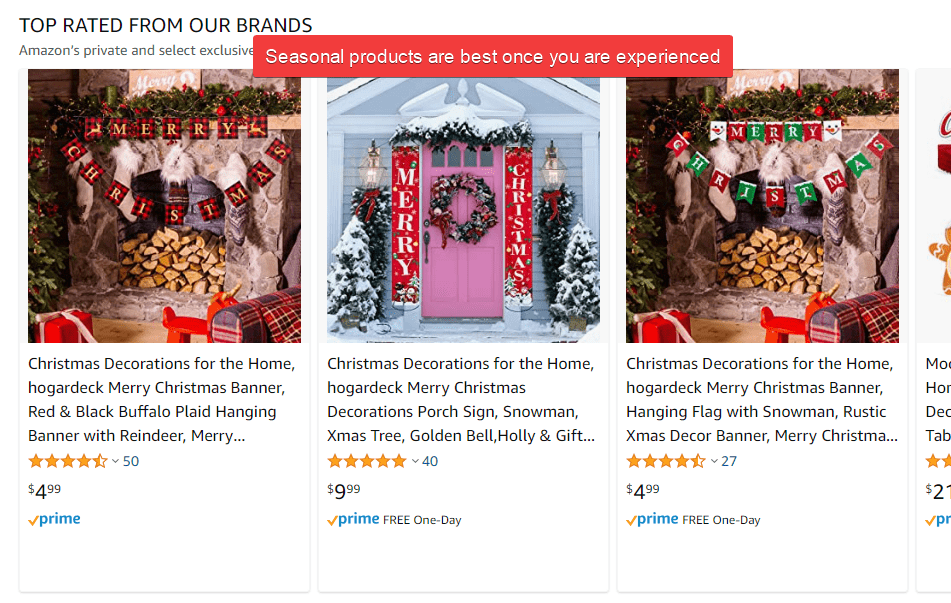This image features a screenshot with a white background. In the upper left-hand corner, the phrase "TOP RATED FROM OUR BRANDS" is displayed in bold, black, all-capital letters. Two lines below that, still in black, it reads "Amazon's private and select exclusive." A red rectangle appears aligned in the center of the screen, partially covering the previous text. The rectangle contains white text stating, "SEASONAL PRODUCTS ARE BEST ONCE YOU ARE EXPERIENCED."

Below this, there are several square photographs arranged horizontally, depicting various Christmas-themed decorations. Visible are three full images and the left edge of a fourth image. The first image showcases a sign saying "Merry Christmas" placed on a fireplace. The second image shows "Merry Christmas" banners on both sides of a pink door. The third image is similar to the first, but with a different "Merry Christmas" banner design. Beneath each photograph is a detailed description in black text.

Further below each description, there are orange stars, representing the rating of the product, and to the right of the stars is a blue number indicating the number of reviews. Two lines further down, the price of each product is displayed in black text, followed by another two lines below where an orange check mark and the word "PRIME" in blue are shown.